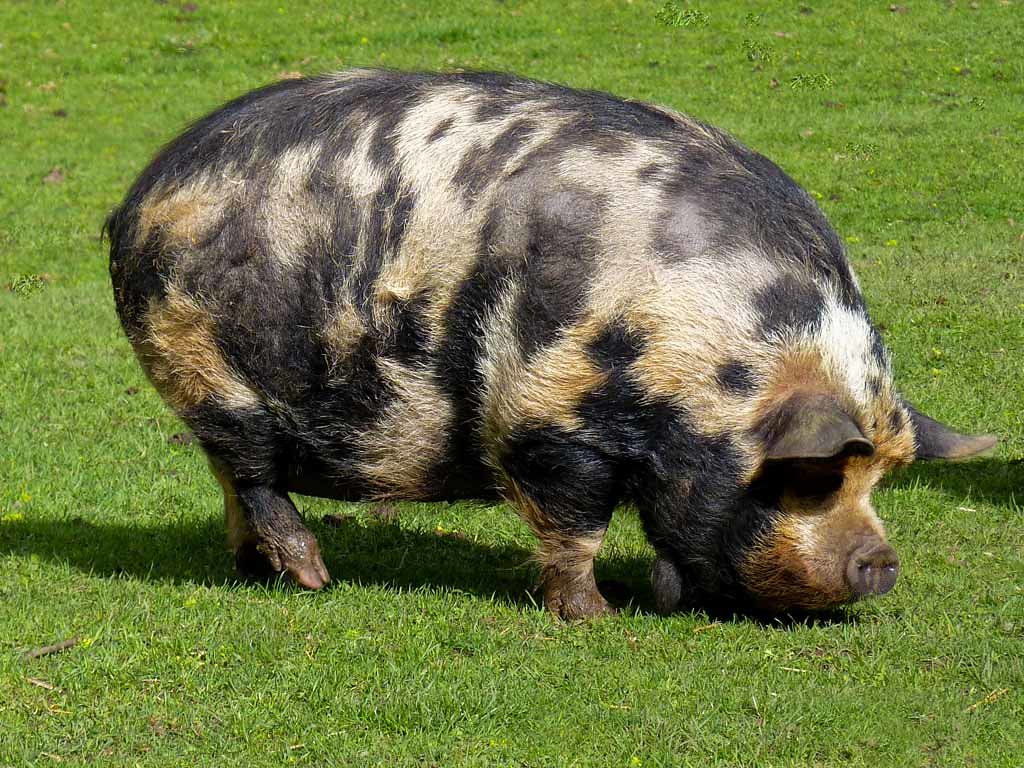This photograph features a very large pig standing in a field of lush green grass that extends to the edges of the photograph. Under a bright, sunny sky, the pig's distinct shadow is cast to the left, indicating the sunny conditions. The pig's head is lowered, with its snout nearly touching the ground, as if about to eat something. It has a dense coat of fur covering most of its body, excluding its ears, the end of its snout, and its hooves. Its fur is a combination of tan, black, and white, creating a mottled pattern, with darker brown patches around its mouth and ears. The entire scene is captured against a backdrop of uninterrupted green grass, emphasizing the pig's imposing size and weight.